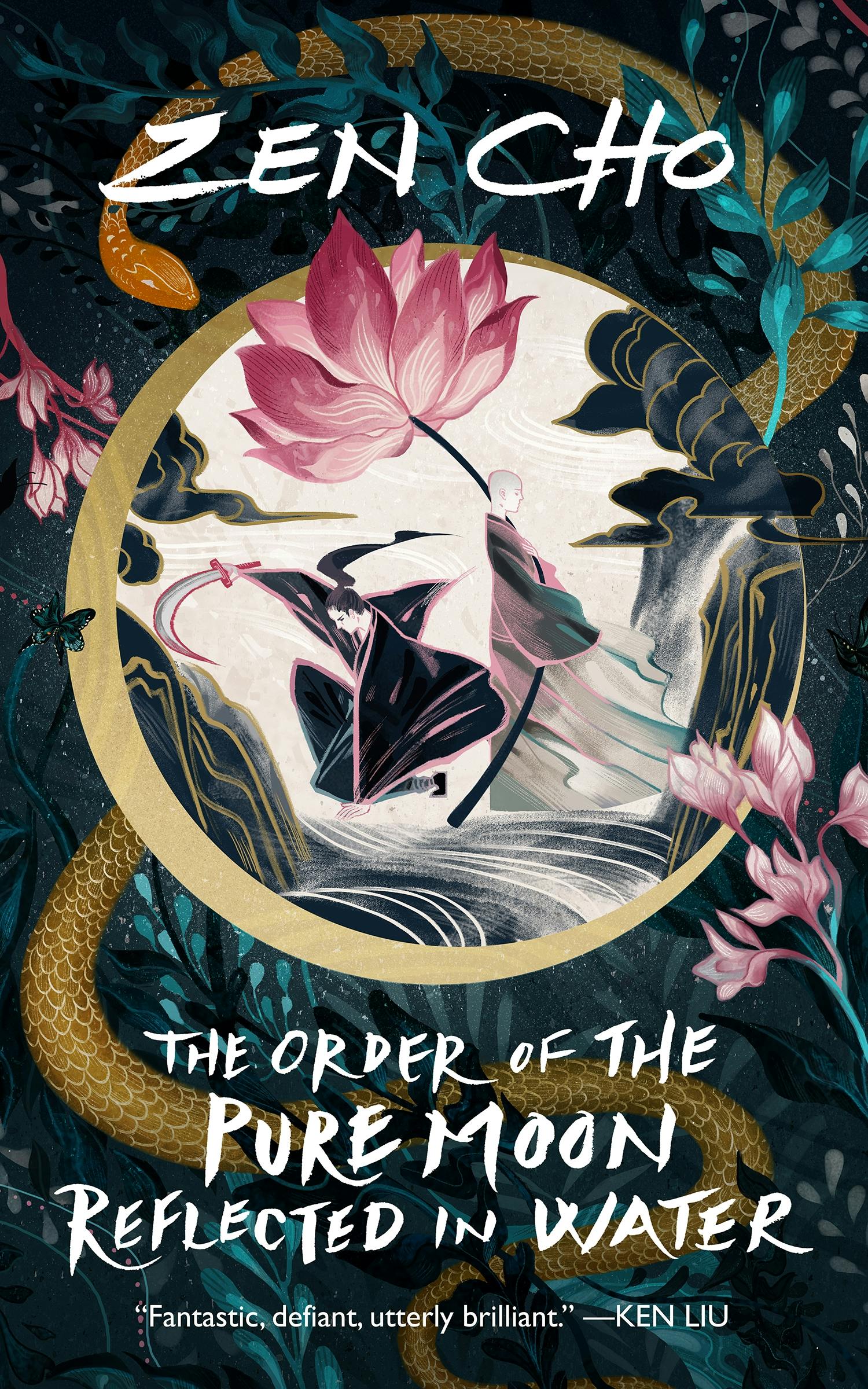This intricate painting features a central circular motif encompassing a dynamic scene. At the heart of the circle is a slender crescent moon, next to which stands a bareheaded monk clad in a flowing black robe that appears to be caught by the wind. The monk holds a large flower with a black stem that stretches across his body; the flower boasts pink, dark pink, and white blossoms. Behind this monk, another monk is depicted in a kneeling position, adorned in a dark cape. Suspended in the air in front of the kneeling monk is a samurai sword. The background within the circle is filled with foreboding black clouds.

Outside the circle, a long snake sinuously makes its way from the bottom to the top of the painting, coiling around as it gazes upon the scene of the two monks. Amidst the snake's path, numerous pink and blue flowers bloom and flourish. Overlaying the entire composition, white brushstroke-like print reads, "The Order of the Pure Moon Reflected in Water." Below this text, an expert's comment praises the artwork, stating, "Fantastic, defiant, utterly brilliant," and is signed by Ken Liu.